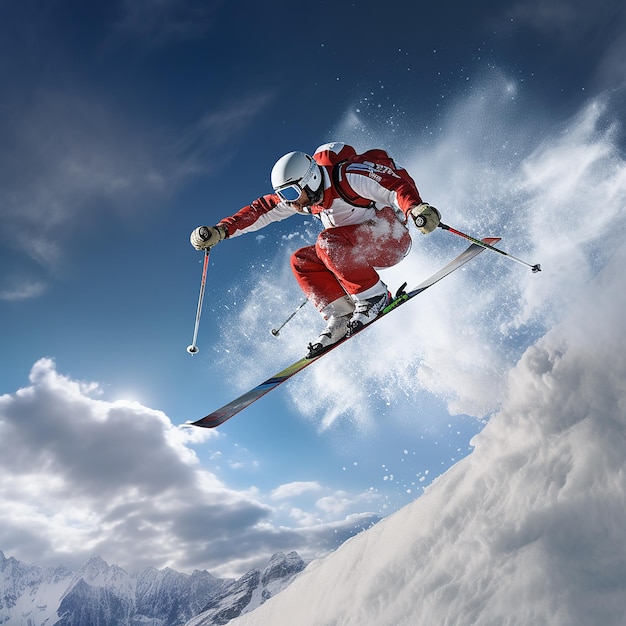In this captivating action shot, a downhill skier, clad in a striking red and white ski suit, soars through the air after launching off a jump or a mountain cliff. The skier, identifiable by a white helmet and matching goggles, grips ski poles in both hands, with a possible extra pole protruding from his back. Uniquely, he balances on a single ski, skillfully managing his descent. The bright day is accentuated by the sun beginning to peak out from behind a fluffy cloud, casting light against a backdrop of majestic mountains and a brilliant blue sky. A dramatic puff of snow trails behind him, indicating the speed and intensity of his jump. The expression on his face and the confidence in his posture capture a moment of pure joy and exhilaration, embodying a passion for the sport amidst a stunning natural setting.